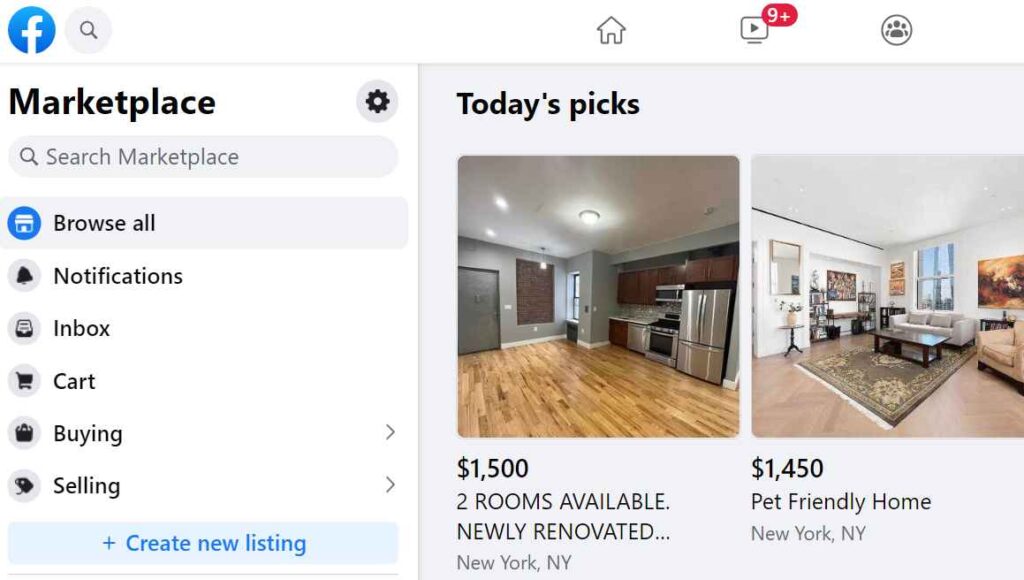The image appears to be a screenshot of the Facebook Marketplace interface. In the top left corner, there is an "F" in a blue circle, which is the Facebook logo. Next to it, there is a magnifying glass icon inside a gray circle, followed by a row of icons: a home icon, a video camera icon with a "9+" notification badge in a red circle, and a group of three people icon within a circle.

On the left side, the word "Marketplace" is displayed along with icons for settings and search. Below this header is a search field labeled "Search Marketplace." Underneath the search field, a vertical menu lists options: "Browse All," "Notifications," "Inbox," "Cart," "Buying," and "Selling." All these options are left-aligned and arranged in a strip along the left side of the interface.

Continuing downward, there is a blue button with darker blue text that says "Create New Listing." On the right side of the interface, a section labeled "Today's Picks" features two photo listings. The first listing on the left shows an image of an interior and reads "$1,500 - Two rooms available, newly renovated, New York, New York." The second listing on the right displays an image of a furnished living room with a couch, and it reads "$1,450 - Pet Friendly Home, New York, New York." 

The image uses a color palette that includes blue, white, gray, red, black, brown, and orange.